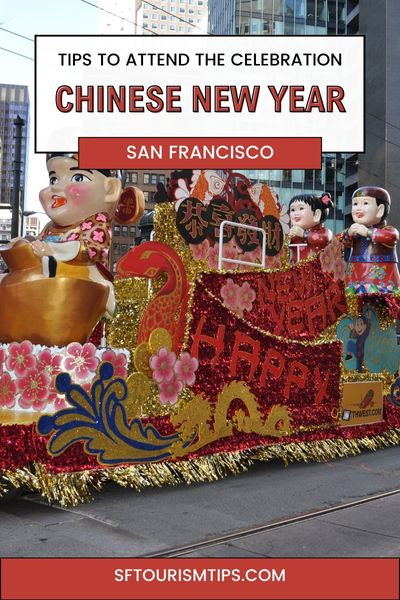The vertical image showcases a vibrant parade float during the daytime, set against the backdrop of modern, 20-30 story buildings in San Francisco. Prominently displayed on the red banner at the top are the words, "Tips to Attend the Celebration Chinese New Year San Francisco," with the URL "sftourismtips.com" at the bottom in white letters. Central to the image is the elaborate float, adorned in gold, blue, and red designs. It features a golden dragon and three large figures with plastic heads, depicting Chinese individuals—one woman at the front and a man and woman towards the back. These figures are set among pink flowers with a white background and three black circles adorned with Chinese writing. The float carries the message "Happy New Year" in striking red letters across various sections. The float rolls over a concrete sidewalk, with possible trolley lines hinting at the San Francisco locale. Sunlight filters through the buildings, casting a warm glow over the celebration scene.